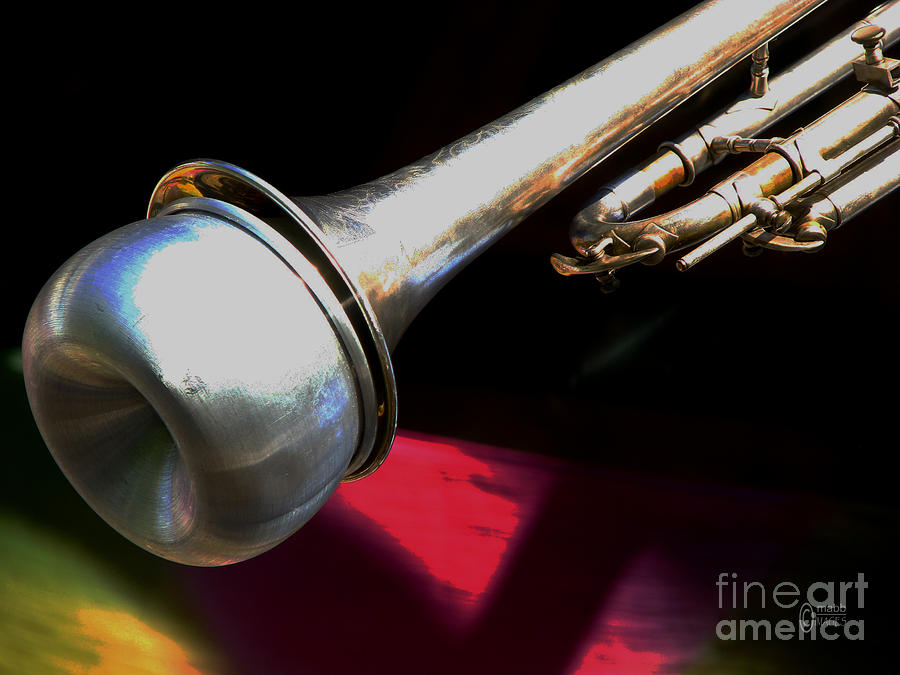In this close-up photograph of a trumpet, we see only its front portion and part of its body. The instrument, appearing silver with hints of brown, prominently features a silver, round-shaped metallic attachment on the main front hole. The background transitions from a predominantly black upper section to a varied lower part with shades of pink, green, yellow, and some darker hues, creating an abstract, almost cosmic scene. This artistic composition gives the appearance that the trumpet is floating over a colorful terrain. Intricate details like the three adjacent valves meant for playing the trumpet are visible. A watermark in the bottom right corner reads "Fine Art America" in light gray against the black backdrop, further emphasizing the artwork’s professional and artistic presentation.